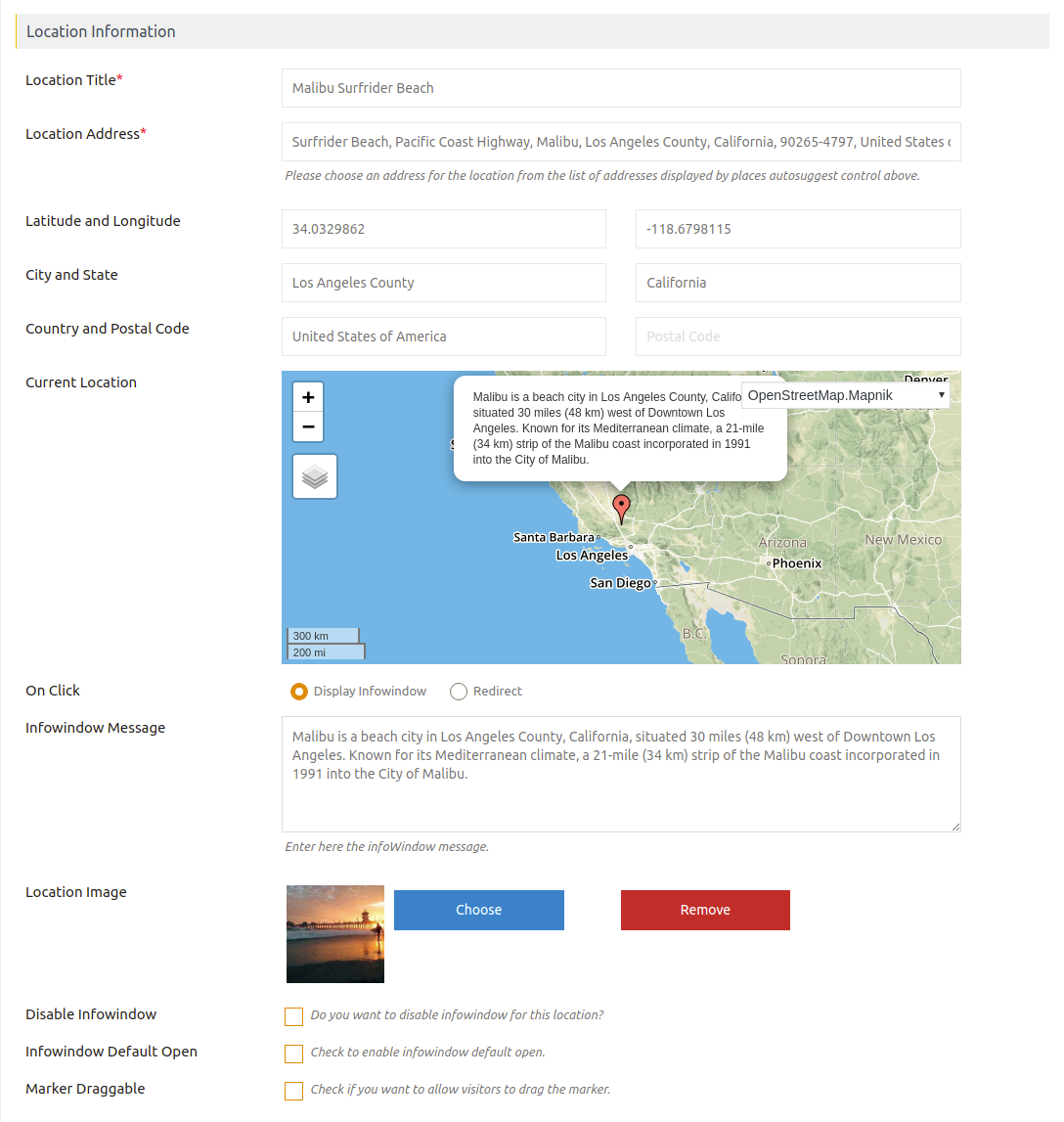This detailed image captures a section of a map-based website focusing on Malibu Surfrider Beach. Positioned in the upper left-hand corner, there is location information encased in a thin gray line. Running vertically down the left-hand side is a list starting with the location title, "Malibu Surfrider Beach." Following this is the address: Surfrider Beach, Pacific Coast Highway, Malibu, Los Angeles County, California, USA. The detailed list continues with latitude and longitude coordinates specific to this locale.

Further down, the city and state are confirmed as Los Angeles County, California, and the country as the United States of America, with the postal code field mentioned as not available. Additionally, it indicates the current location. To the right of this comprehensive list, there's an embedded map featuring a highlighted marker at Malibu with an info window stating, "Malibu is a beach city in Los Angeles County, California."

Below this map snippet, options such as "Disable Info Window," "Info Window Default Open," and "Marker Draggable" are visible, providing an array of customizable features for the user's interaction with the map. This detailed caption encapsulates all textual and visual elements within the image, focusing on the geographical and interactive specifics of the Malibu Surfrider Beach location within the map interface.